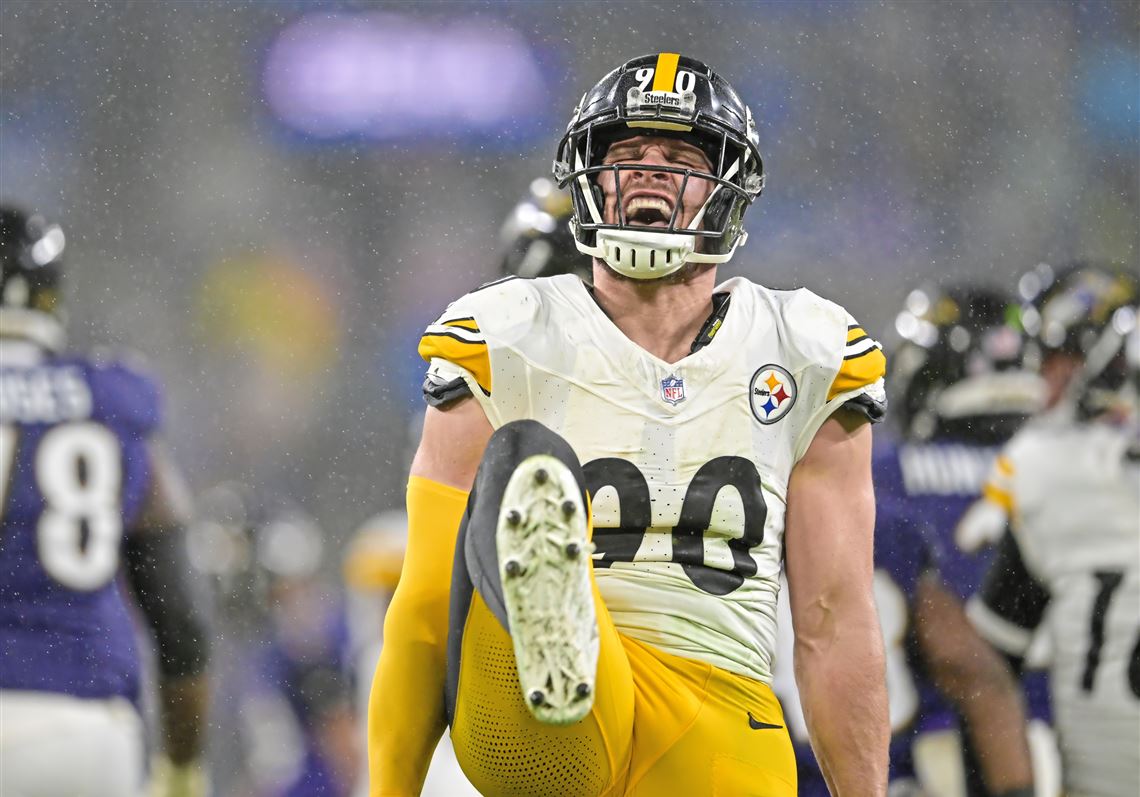This photograph captures TJ Watt, a defensive end for the Pittsburgh Steelers, in action during a game where it appears to be snowing, as evidenced by the small white dots falling around him. Watt is mid-kick with his right leg lifted high, showcasing the bottom of his cleated shoe and white sock. 

He dons a white jersey with the number 90 prominently displayed on his chest, although the view is partially obscured as his shirt twists with his movement. His gold pants feature a visible Nike swoosh, and a yellow compression-like arm sleeve adorns his right arm. Watt is also wearing a black helmet, distinguished by a yellow stripe down the center and the number 90 in white. 

To the left and right of Watt, other players are visible, some in white jerseys and others in dark purple ones, suggesting a diverse team setting. A player to the left displays the number 8 on his uniform. Above Watt’s left arm near his shoulder, the Steelers logo is noticeable, characterized by its three diamond shapes in yellow, red, and blue.

Watt's mouth is agape, possibly indicating the intensity of the moment or an expression of exertion or pain. The scene is a vivid snapshot of the dynamic and raw energy of the game.